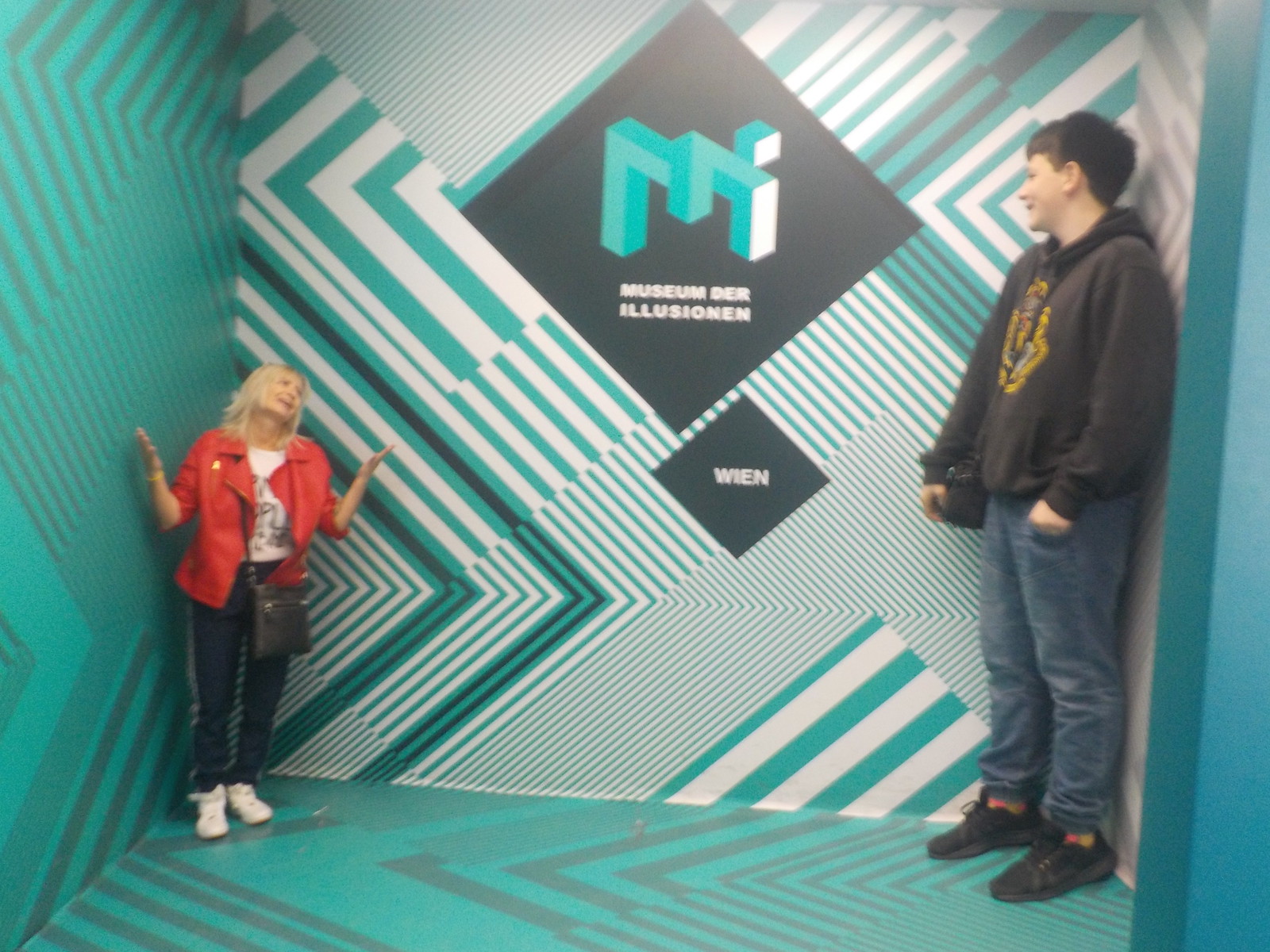In this photograph taken at the Museum der Illusionen, an indoor setting designed to play with perception, a visual trick makes a young boy appear much larger than an older woman. The boy, positioned on the right side of the room, is dressed in a dark sweatshirt hoodie, blue jeans, and black shoes. He has short brown hair and is smiling down at the woman. The woman, positioned in the left corner, is wearing a red jacket over a white shirt, blue jeans, white sneakers, and has a black purse slung across her chest. She has blonde hair and her hands are raised in a gesture that suggests surprise or confusion. The room's walls are adorned with geometric patterns in greens, grays, teal, and black, enhancing the illusion. The writing on the back wall reads "Museum der Illusionen," indicating this is a place dedicated to optical illusions. The room's design makes the boy appear like a giant compared to the diminutive woman, showcasing a classic example of perspective illusion.